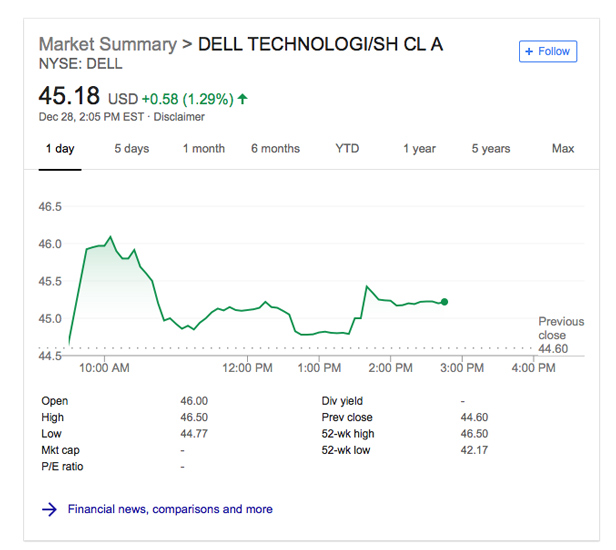Screenshot of Dell Technologies Market Summary on the NYSE platform. The image features a prominent square with a gray border and a white background. At the top, "Market Summary" is clearly labeled alongside "Dell Technologies (NYSE: DELL)." On the top right, a blue-bordered rectangle marked "Follow" is visible.

The stock price is displayed prominently in bold print as $45.18 USD. Beneath this, a green arrow indicates a positive movement, showcasing an increase of $0.58 or 1.29%. The date of this data is also present.

The center of the screenshot features a detailed line graph depicting the stock's performance. The graph, formed with a green line, shows significant fluctuations: it initially spikes upward and then curves around. The timeline at the top allows viewing from one day to a maximum range of up to five years, while the vertical axis on the left marks the stock's value.

Beneath the graph, benchmark statistics are organized in two columns, each listing various financial metrics alongside their corresponding values. At the bottom, a blue arrow pointing to the right indicates additional options for "Financial News," "Comparisons," and more information.